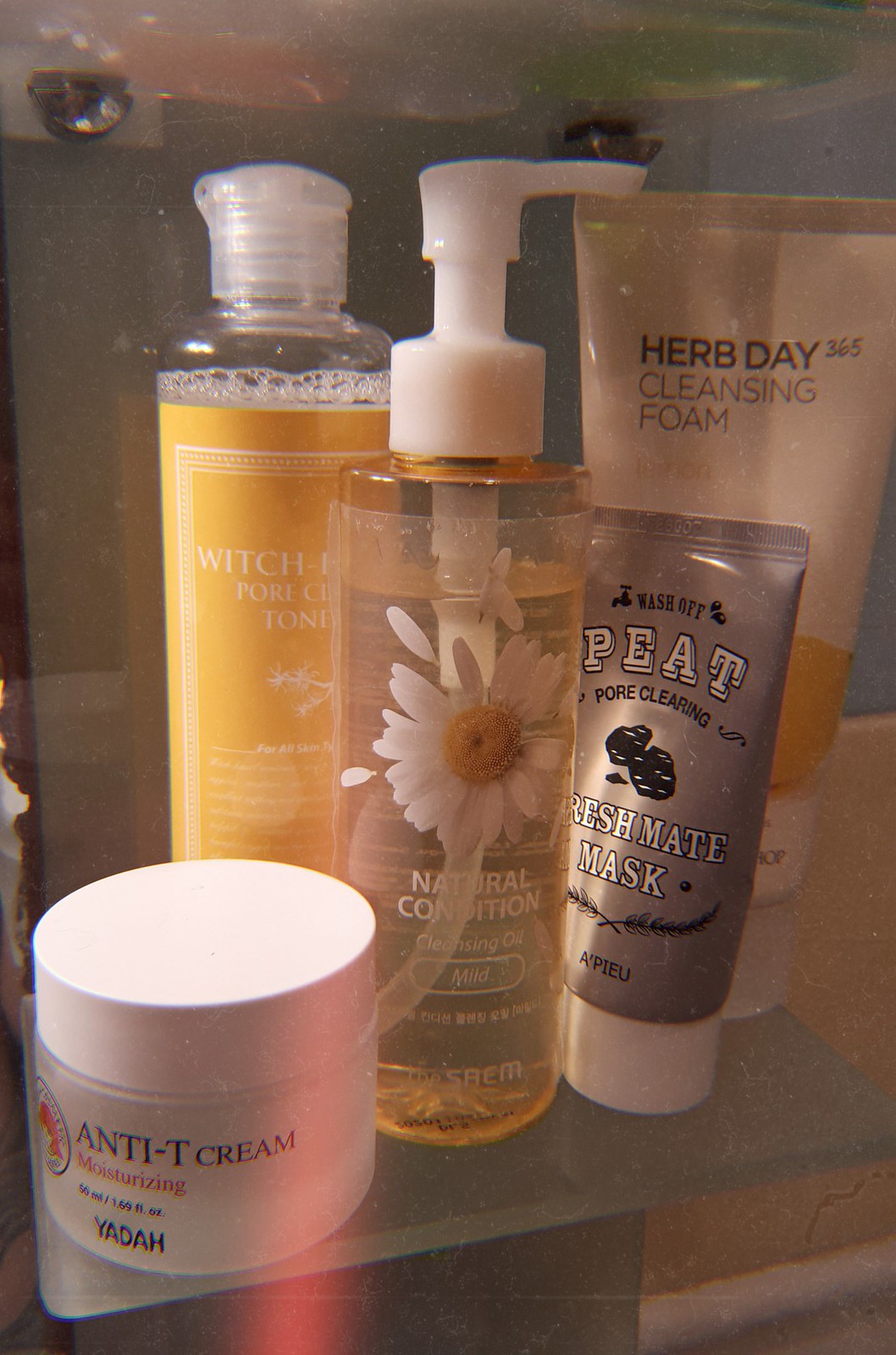This photograph captures a meticulously arranged display of skincare products, either in a personal bathroom or a retail setting, under soft indoor lighting without the use of a flash. 

In the lower left corner, prominently featured in the foreground, is a white plastic jar with a screw-off lid, labeled "Anti-Tea Cream." The jar also mentions "moisturizing" properties and has other small text detailing the weight, which is too small to be legible. The brand name "Yadah" is also displayed.

Directly behind this jar is a clear plastic bottle with a pump top, labeled "Natural Condition" and adorned with an image of a white daisy losing some of its petals, which appear to be floating away. The bottle is mostly filled with a clear, yellowish fluid.

Next to these, positioned a bit further back, is another clear plastic bottle featuring a yellow label with the words "Witch Pore Toner," indicating that it is likely a witch hazel toner. This bottle is nearly full.

In the lower right foreground, there is a plastic squeeze tube labeled "Peat Pore Cleaning Fresh Mate Mask." This tube resembles a toothpaste container and is resting on its white lid.

Behind this, there is a larger tube labeled "Herb Day Cleansing Foam." This white plastic container, decorated with yellow designs, is also resting on its lid.

All these items are neatly placed on what appears to be a glass shelf. A hint of another glass shelf above adds to the organized and clean aesthetic of the display.